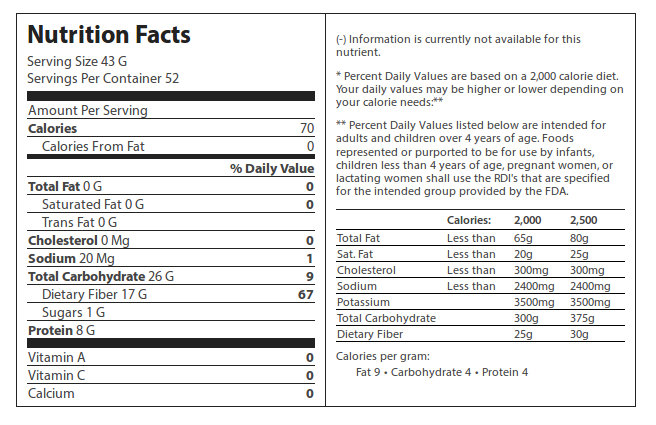This image appears to be a detailed screenshot of a generic nutrition facts label, typically found on the packaging of food products such as cans of soup or other grocery items. The entire label is set against a white background with various sections and information arranged in a structured format. 

At the top left, the heading "Nutrition Facts" is prominently displayed in bold black text. Below this heading, the label provides specific information about serving size, with "Serving Size 43g" and "Servings Per Container 52" clearly listed. The data includes key nutritional details such as total fat, calories, cholesterol, and sodium, with certain items like "Total Fat" and "Calories" emphasized in bold text to highlight their importance.

To enhance readability, black separator bars are used on the left side to organize different sections of information. The central part of the label contains detailed content on daily values and percentages, explaining what these nutritional metrics mean in the context of a daily diet.

On the right side, additional notes are provided to clarify certain terms and values, including a breakdown of calories derived from various nutrients. A vertical separator in the middle divides the main nutrition facts from this explanatory section.

The entirety of the information is encased within a subtle gray border, giving the label a complete and structured appearance. This label represents a standard template and is likely used for illustrative or informational purposes, rather than depicting a specific product.